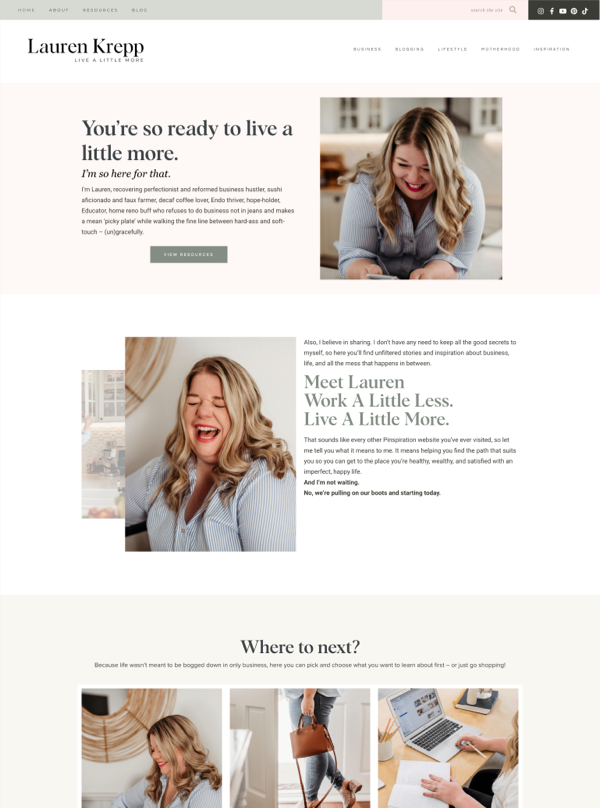The image depicts a blog-style website featuring multiple images and text elements. At the top left corner, the navigation menu includes links labeled "Home," "About," "Resources," and "Blog." Adjacent to it, a pink search bar titled "Search the Site" is prominently displayed, along with icons for social media platforms including TikTok, Facebook, and YouTube, plus two additional, unidentifiable icons.

The site header is divided into two parts: on the left, it reads "Lauren Krimp, Live a Little More," while on the right, it categorizes content into "Business," "Blogging," "Lifestyle," "Motherhood," and "Inspiration." Below this, a pink-colored box contains an inviting message: "You're so ready to live a little more. I'm so here for that. I'm Lauren, recovering perfectionist and reformed business hustler, sushi aficionado, and faux farmer, decaf coffee lover, endo-thriver, hope-holder, educator, home-reno-buff, who refuses to do business not in jeans and makes a mean picky plate while walking the fine line between hard-ass and soft-touch, ungracefully. View Resources."

An image of a woman, presumably Lauren, showcases her in a blue-striped shirt, smiling broadly with blonde hair and red lipstick. Beneath this image, another text section reads: "Also, I believe in sharing. I don't have any need to keep all the good secrets to myself. Here you'll find unfiltered stories and inspirations about business, life, and the mess that happens in between. Meet Lauren, work a little less and live a little more. I'm not waiting. No, we're pulling on our boots and starting today. Where to next? Because life wasn't meant to be bogged down in only business."

The page concludes with an invitation to "pick and choose what you want to learn about first, or just go shopping," accompanied by three more images below this text.